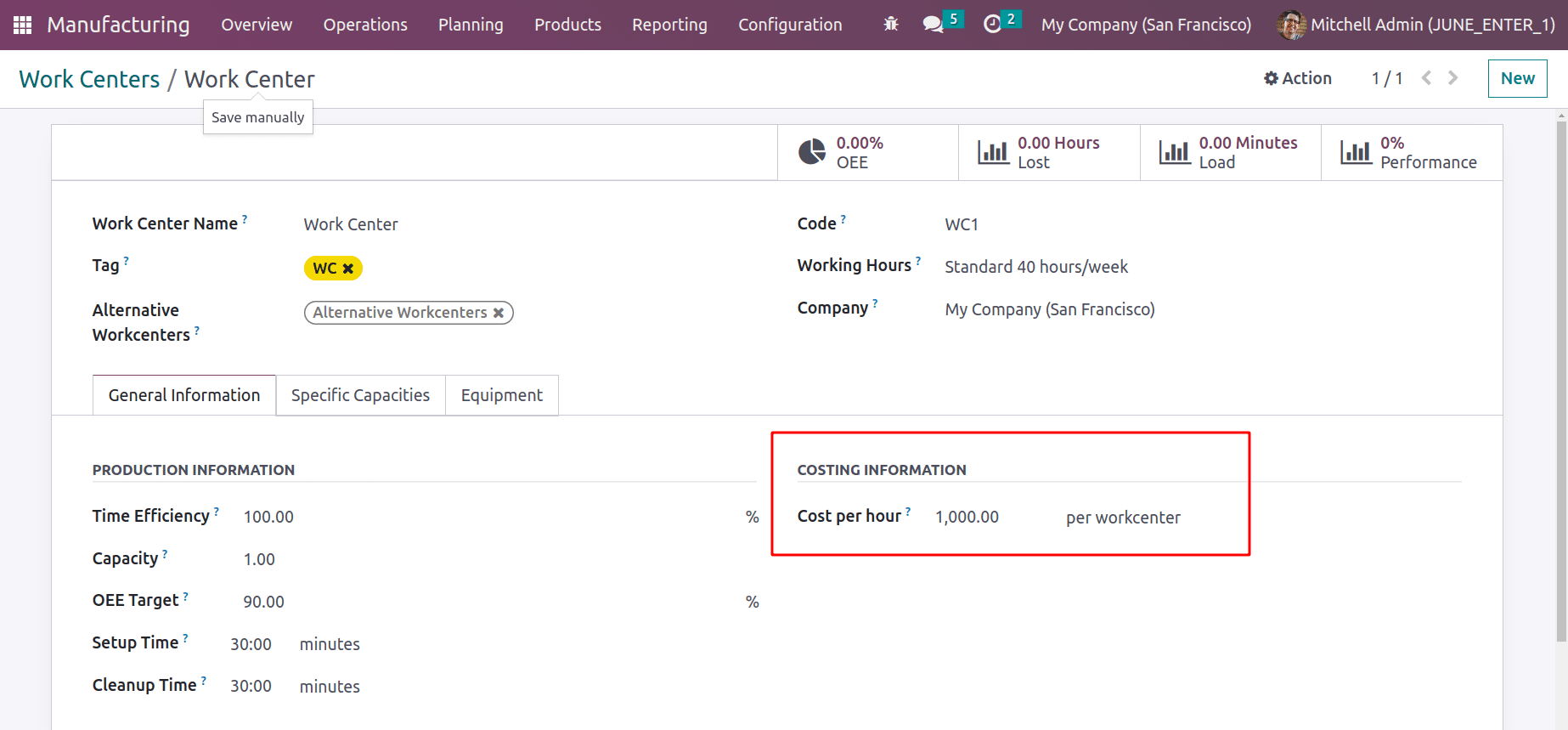This image showcases a detailed view of a web page interface, likely used for managing manufacturing operations.

At the top left of the page, there's a navigation bar with multiple tabs labeled from left to right: Manufacturing, Overview, Operations, Planning, Products, Reporting, and Configuration. Following these tabs, there are three icons in sequence: a bug icon, a comment icon, and a clock icon.

Next to these icons, the text "My Company (San Francisco)" is displayed. Adjacent to this text, there is a profile image of a person's face. On the right, the profile name "Mitchell Admin" is shown, followed by the text in parentheses: (June_enter_one).

Below this top section, on the left side of the page, there is a section labeled "Work Centers / Work Center Save Manually." Beneath this header, the information is displayed in a structured format: "Work Center Name, Work Center Tag (WCX), and Alternative Work Centers."

Three tabs are located below this section, with labels from left to right: General Information, Specific Capacities, and Equipment. Further down, there is a section titled "Production Information," next to which the text "Time Efficiency" is visible.